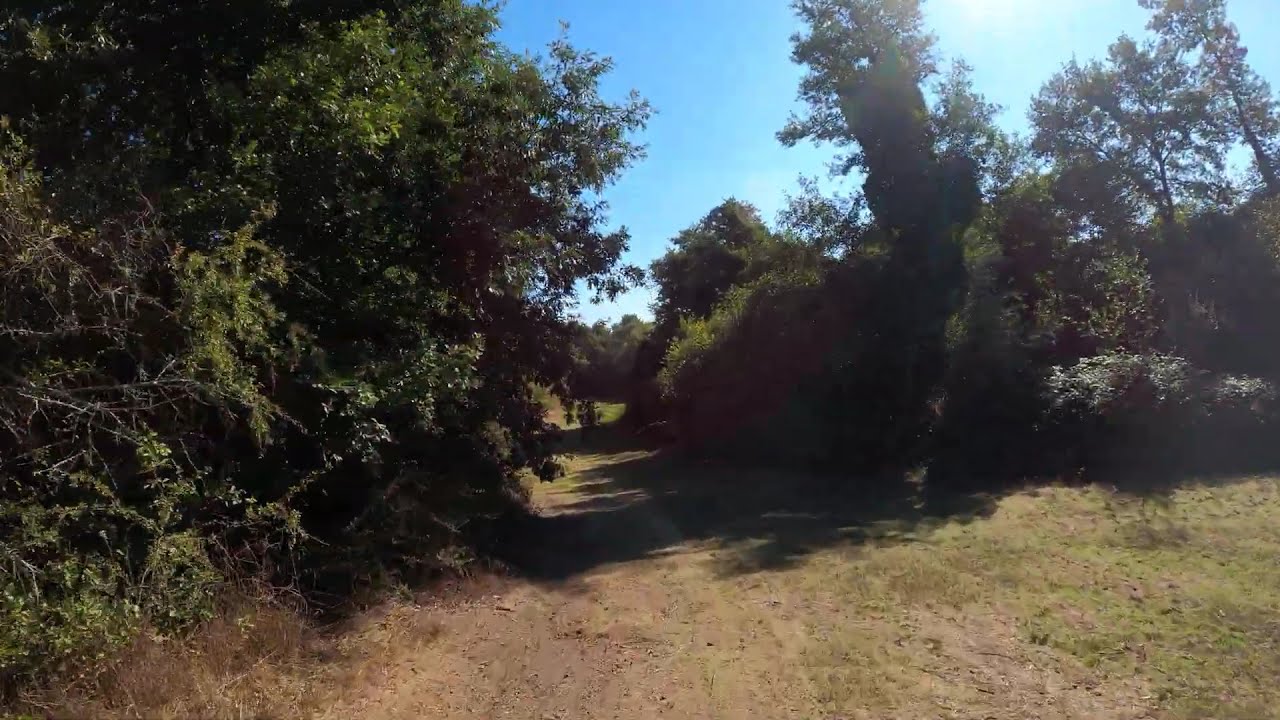The photo depicts a serene, green environment, likely a nature preserve, featuring an unpaved, brown trail that meanders through lush fields of green grass. On the left of the path, the robust trees are dense and leafy, obscuring much of the sky, while the trees to the right are shorter, allowing glimpses of the blue, cloudless sky. A wide-trunked tree stands prominently among the shorter trees. The sun beams down from the top right, casting a warm glow over the scene. No cars or electrical wires disrupt the tranquility. In the distance, two people walk along the lightly trodden trail, hinting that it may be popular with hikers. The picture captures the peaceful essence of untouched nature, with abundant green foliage and a clear, inviting sky.